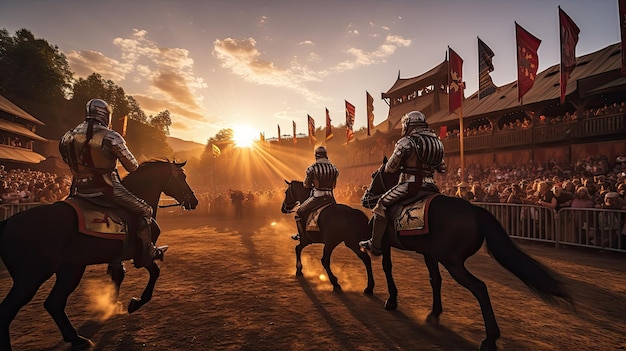In this richly detailed scene, we observe a captivating work of art depicting three knights, clad in gleaming steel armor, astride their brown steeds. The composition is wider than it is tall, perhaps one and a half to two times in width. The knights, their backs to us, appear to be riding towards a mesmerizing horizon where the sun is either setting or rising, casting a golden hue over the landscape and illuminating the dirt ground beneath them. Flanking the dirt pathway, crowds of onlookers cheer enthusiastically from behind modern metal fencing, suggestive of a Renaissance festival or similar historical reenactment.

The intricate details of the scene are further accentuated by the colorful banners adorning the surroundings. A variety of flags, including a red one, a black and white one, a red flag with yellow and green flowers, and another red flag with indistinct symbols, flutter in the upper right corner. Additional flags are visible towards the top of the image, adding to the festive atmosphere.

Each knight's horse is draped in luxurious blankets with silver trim and possibly accents of red, enhancing their regality. A raised terrace along the left and right sides of the image provides a vantage point for the spectators, who eagerly anticipate the knights' performance. The image, steeped in medieval elements yet featuring hints of modernity, captures the timeless allure of chivalric tournaments and the enduring excitement they generate among audiences.